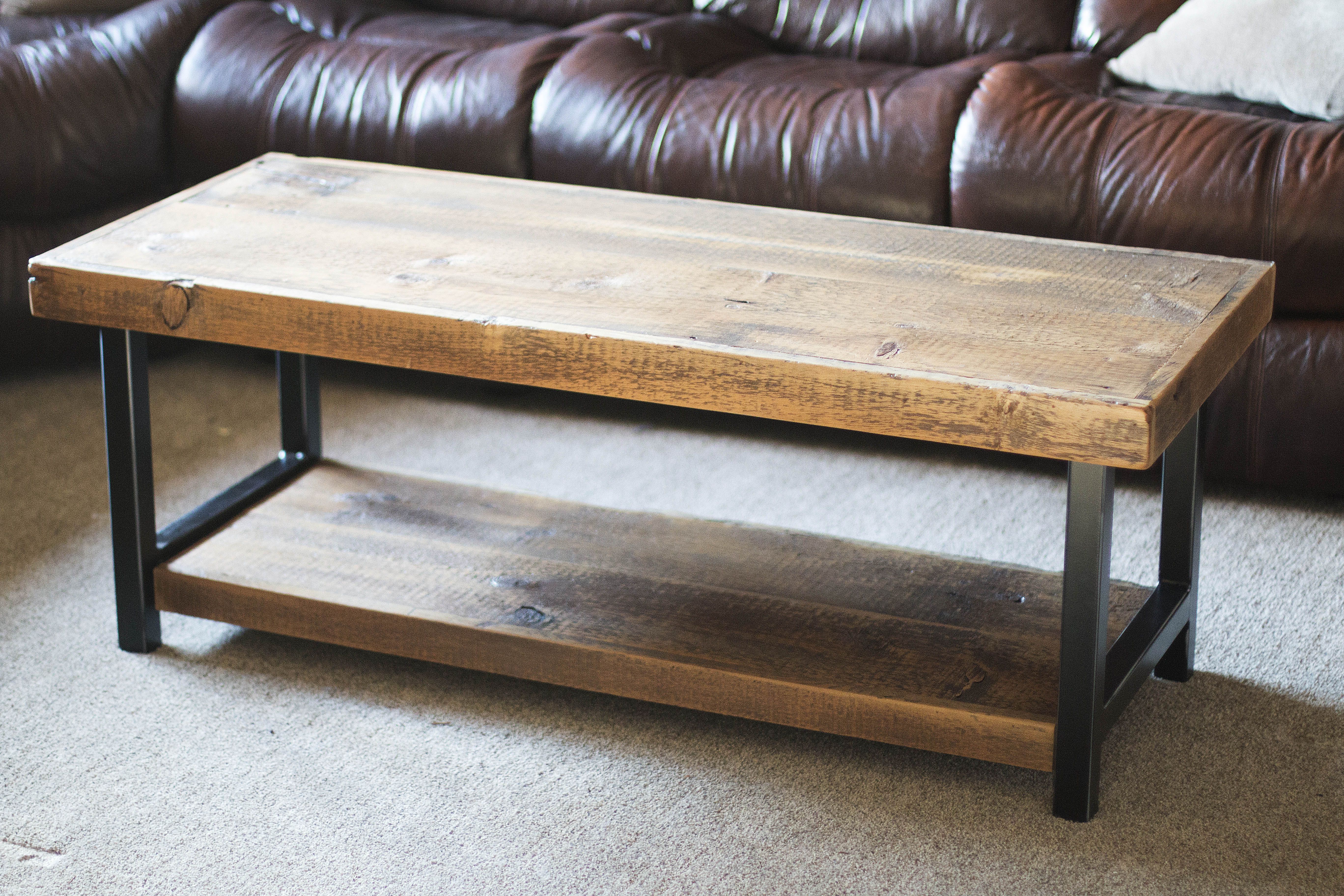The photograph captures a detailed scene of a living room, focusing on a distinct wooden coffee table at its center. The table is constructed from two wooden planks - a larger rectangular surface on top and a similarly shaped bottom shelf, perfect for additional storage. It's held up by four sturdy black metal legs. The wood of the table is marked with multiple dark knots, adding to its rustic charm. This table sits on a carpet with short, tan, or whitish fibers, blending subtly into the setting. Behind the coffee table is a large brown leather couch with individual seats, characterized by noticeable wrinkles in the leather. One of the plush fluffy cushions on the sofa features a white pillow, prominently positioned to the right. The entire scene exudes a cozy and inviting atmosphere, with the coffee table and the leather couch serving as the focal points.